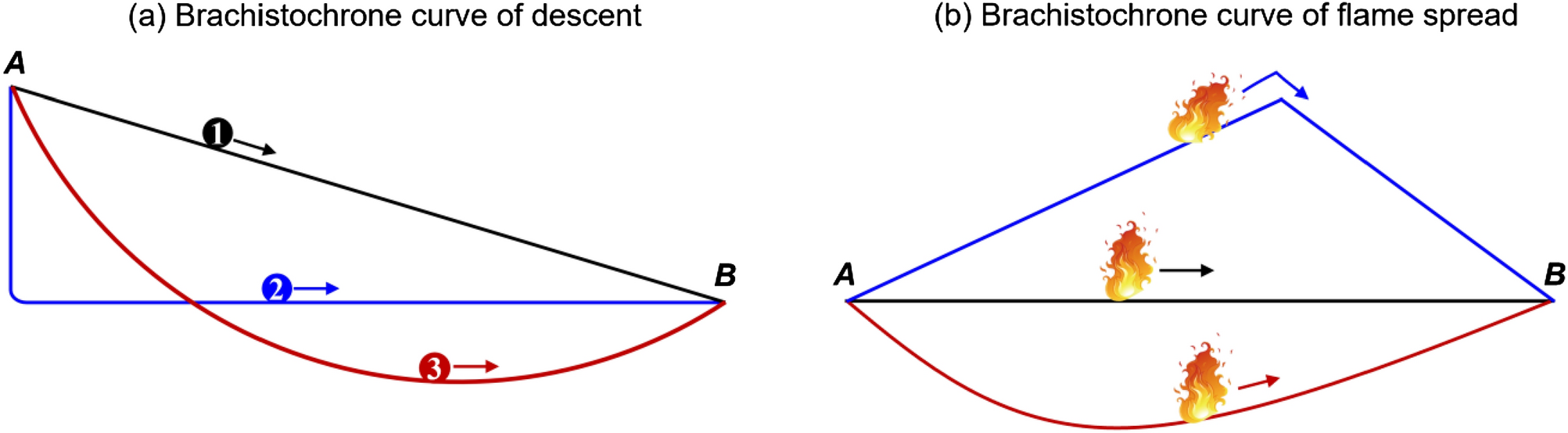This detailed diagram illustrates two separate concepts under the heading of 'Brachistochrone'. 

On the left side, under the label 'A', the diagram explains the 'Brachistochrone curve of descent'. At the top, labeled 'A', it features a thin, right-angled triangle with a black hypotenuse and a blue vertical leg. An arrow labeled '1' points to the black hypotenuse, while another arrow labeled '2' indicates the blue vertical leg extending to the point 'B' at the bottom. A red curved line, marked with an arrow labeled '3', descends from 'A' to 'B'.

On the right side, the diagram depicts the 'Brachistochrone curve of flame spread'. Shaped like an inverted blue triangle with a flat base and apex labeled 'A', it details the spread pattern of flames. An arrow at the top indicates 'A', with flames depicted alongside the arrow. A central black line with flames is labeled with an arrow pointing to 'B'. Finally, a red line curves in a semi-circular manner at the bottom, with flames and a red arrow positioned centrally.

This well-annotated diagram provides a visual comparison of the Brachistochrone curve in the contexts of both descent and flame spread, marked with clear geometric and color-coding elements to distinguish the different paths.